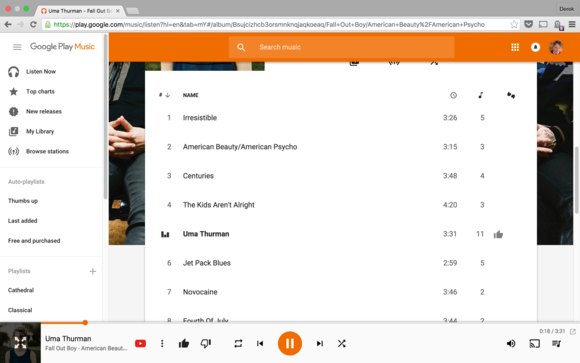Screenshot of a user interface on Google Play Music displayed on a MacBook. The interface includes the characteristic red, yellow, and green window control buttons in the upper left-hand corner, with the yellow dot grayed out. The user is currently listening to "Uma Thurman" by Fall Out Boy, and the interface shows the album "American Beauty/American Psycho," featuring songs such as "Irresistible," "American Beauty/American Psycho," "Centuries," "The Kids Aren't Alright," "Uma Thurman," "Jetpack Blues," "Novocaine," and "Fourth of July."

In the upper left corner of the interface, the Google Play Music logo is displayed alongside a hamburger menu. Tabs for "Listen Now," "Top Charts," "New Releases," "My Library," and "Browse Stations" are organized horizontally. Auto-generated playlists include "Thumbs Up," "Last Added," "Free and Purchased," and a few custom playlists labeled "Cathedral" and "Classical."

In the upper right corner, the user is logged in. Their profile picture depicts an older white male with medium-length hair. Next to the profile picture is a small star button and the Google Apps menu, represented by a nine-square icon. Adjacent to these are icons for volume control, casting to a device, and the music queue.